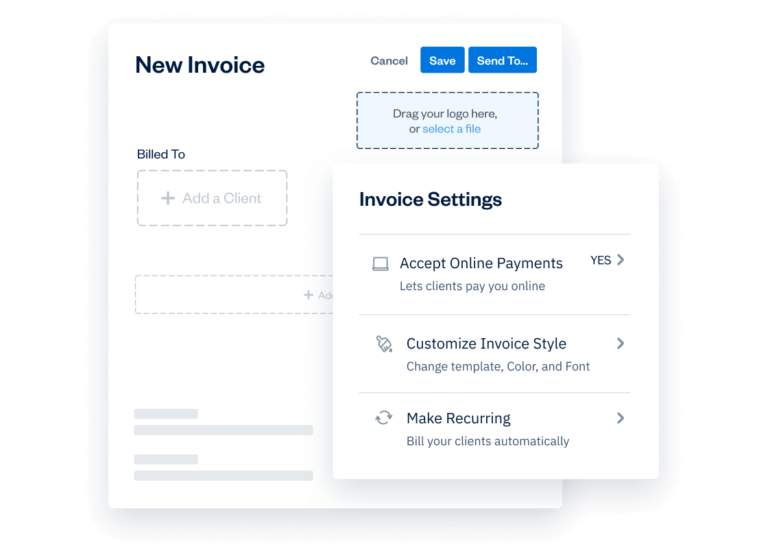The image showcases an interface for creating and managing invoices. 

In the background, there is a larger "New Invoice" box with a pristine white backdrop. The text is primarily in black, with accents provided by blue buttons. In the upper left corner of this box, "New Invoice" is prominently displayed. Adjacent to this on the right, there is a "Cancel" button followed by two blue action buttons labeled "Save" and "Send To."

Below these buttons, there is a light blue, dotted-bordered box with the instruction "Drag your logo here or select the file." 

On the left side of the "New Invoice" box, there is a "Bill To" section featuring an "Add a Client" field, which is currently grayed out, indicating it is not active or clickable.

In front of this "New Invoice" box, occupying a central position, there is a slightly smaller "Invoice Settings" box, which appears in the foreground. This box outlines various settings options:
- "Accept Online Payments": This option is highlighted and accompanied by the statement "Let clients pay you online."
- "Customize Invoice Style": This outlines the possibility to change the template, color, and font of the invoice.
- "Make Recurring": This option allows for automatic billing of clients.

Overall, this image seems to display a user-friendly guide to navigating the invoice creation and settings interface, detailing how users can personalize their invoices and streamline the payment process.